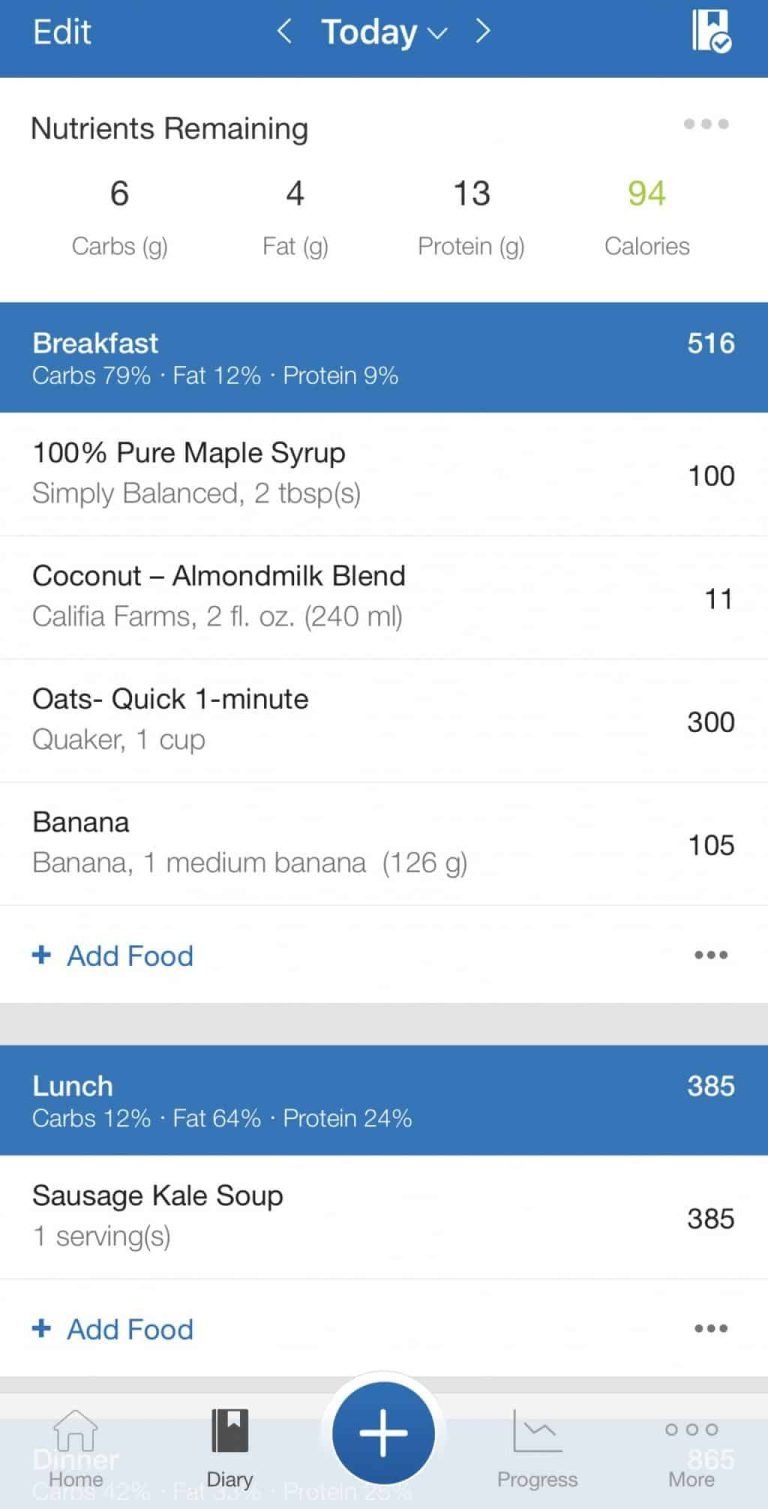This image shows a dietary tracking application with three distinct sections. Each section has a blue background with white subheadings. 

1. **Today's Edit:**
   - Under this section, the remaining nutrients are displayed:
     - Carbohydrates: 6 grams
     - Fats: 4 grams
     - Calories: 94 (highlighted in green)

2. **Breakfast:**
   - Nutrient distribution:
     - Carbohydrates: 79%
     - Fats: 12%
     - Protein: 9%
   - Food items listed:
     - 100% Pure Maple Syrup (Simply Balanced): 2 tablespoons (100 calories)
     - Coconut Almond Milk (Almond Milk Blend, Califia Farms): 240 milliliters (11 calories)
     - Quaker Quick One Minute Oats: 1 cup (300 calories)
     - Banana: 1 (115 calories)
   - Total calories for breakfast: 516

3. **Lunch:**
   - Nutrient distribution:
     - Carbohydrates: 12%
     - Fats: 64%
     - Protein: 24%
   - Food item listed:
     - Sausage Kale Soup: 1 serving (285 calories)
  
At the bottom of the application interface, there are navigation options:
   - **Home:** Positioned at the bottom left
   - **Diary**
   - **Add:** Centered, represented by a white plus sign on a blue circle
   - **Progress**
   - **More:** Positioned at the bottom right